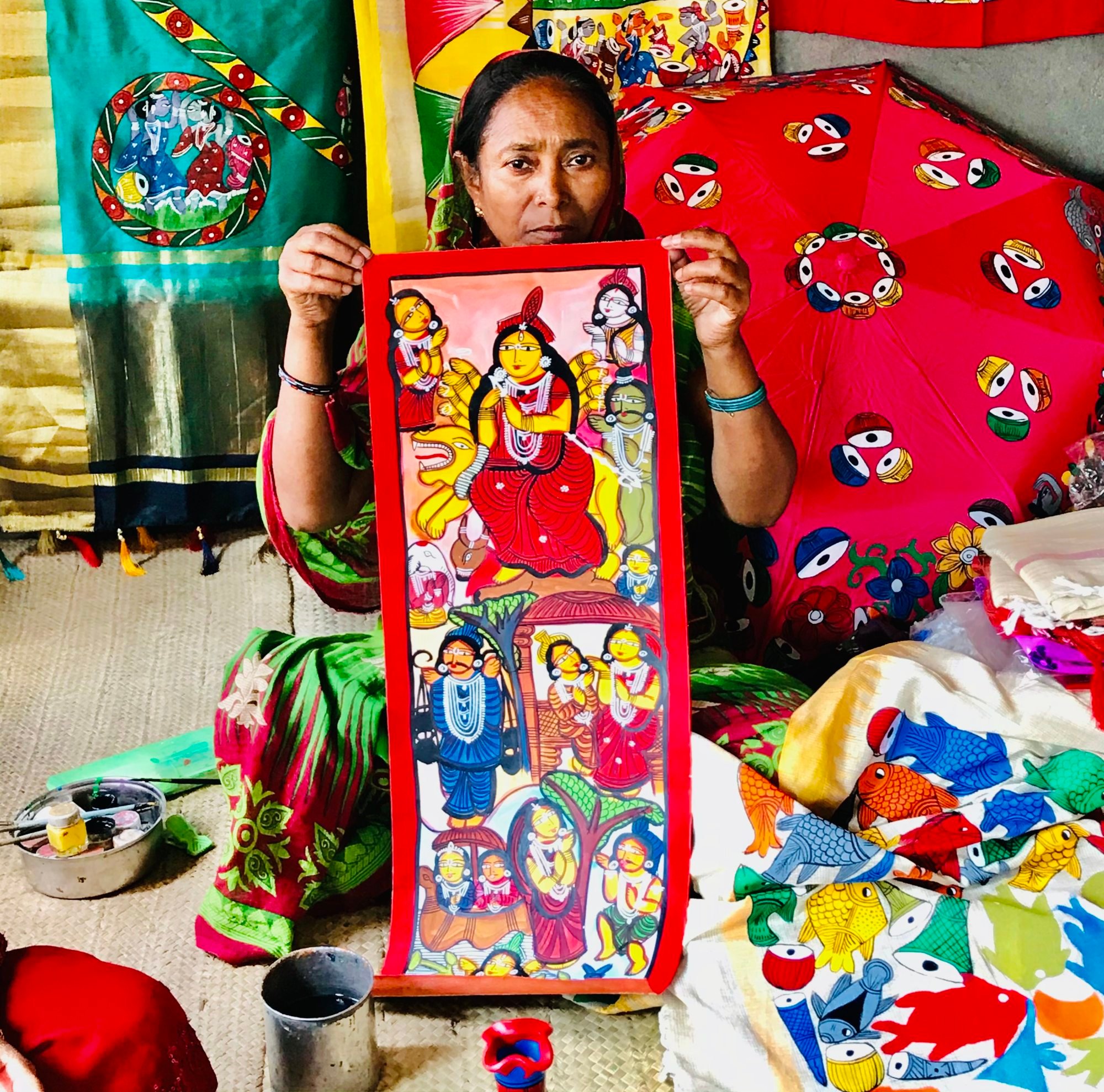A captivating indoor photograph showcases a woman with striking black hair, dark skin, and deep black eyes. She adopts a neutral expression while holding up an intricately detailed tapestry. Adorning her wrists are two wristbands: one is a vivid blue, and the other is black featuring white stripes. She wears a dress that stands out with its green patterns set against a red background.

The tapestry she presents is a vibrant and complex piece of art. Central to it is another woman, seated and dressed in a rich red dress, her black hair cascading around her. Flanking this central figure are multiple characters adorned in varying patterns, adding a layer of diversity and richness to the scene. Below them stands a man in a blue robe, cradling something in his arms, which adds a narrative depth to the tapestry. The bottom section portrays two women amongst various other figures, making the tapestry a multi-faceted portrayal of life and culture.

The setting of the photograph is illuminated by natural light, enhancing the colors and details in the scene. The background is a tapestry of its own, filled with various sheets and items. Notably, one sheet features patterns of fish, contributing to the aquatic theme. Additionally, an umbrella embellished with drum images and other tapestries scattered around add to the cultural and artistic ambiance of the room.